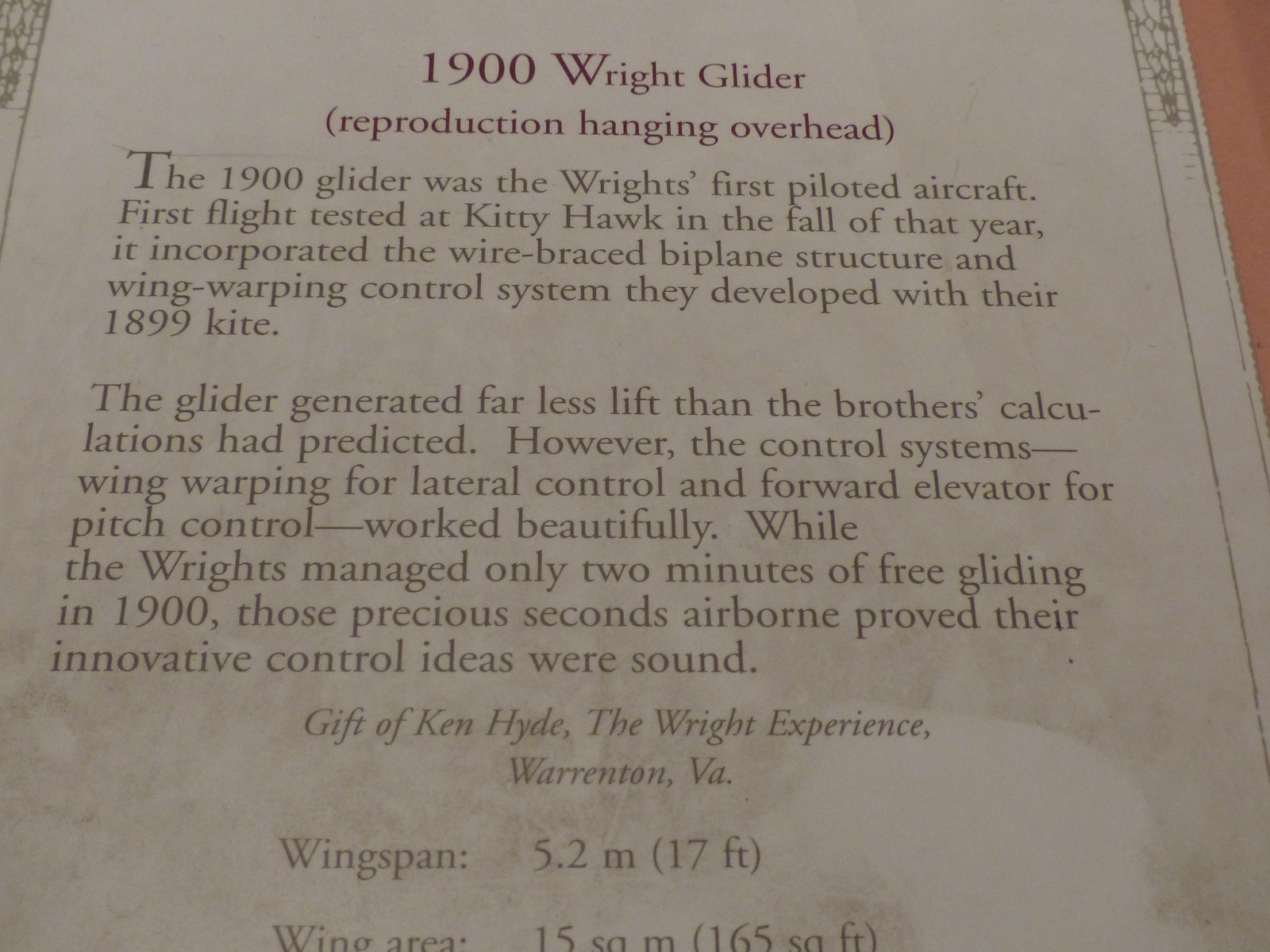This image displays a museum plaque affixed to a wall, possibly peach-colored, describing the 1900 Wright Glider. The top of the white plaque prominently features the title in dark red or brownish-purple text: "1900 Wright Glider (reproduction hanging overhead)." Below, two well-detailed paragraphs outline the significance of the Wrights' pioneering aircraft, which was their first piloted glider, flight-tested at Kitty Hawk in the fall of 1900. It incorporated the advanced wire-braced biplane structure and wing-warping control system developed from their 1899 kite design. Notably, the glider produced less lift than predicted by the brothers' calculations. Nevertheless, the control systems, utilizing wing warping for lateral control and a forward elevator for pitch control, functioned effectively. Although the Wrights achieved only two minutes of free gliding that year, these brief moments were crucial as they validated the innovative control concepts. At the bottom of the plaque, the information credits "Ken Hyde, The Wright Experience, Warrington, VA," and specifies the glider's wingspan of 5.2 meters (17 feet) and wing area of 15 square meters (165 square feet).